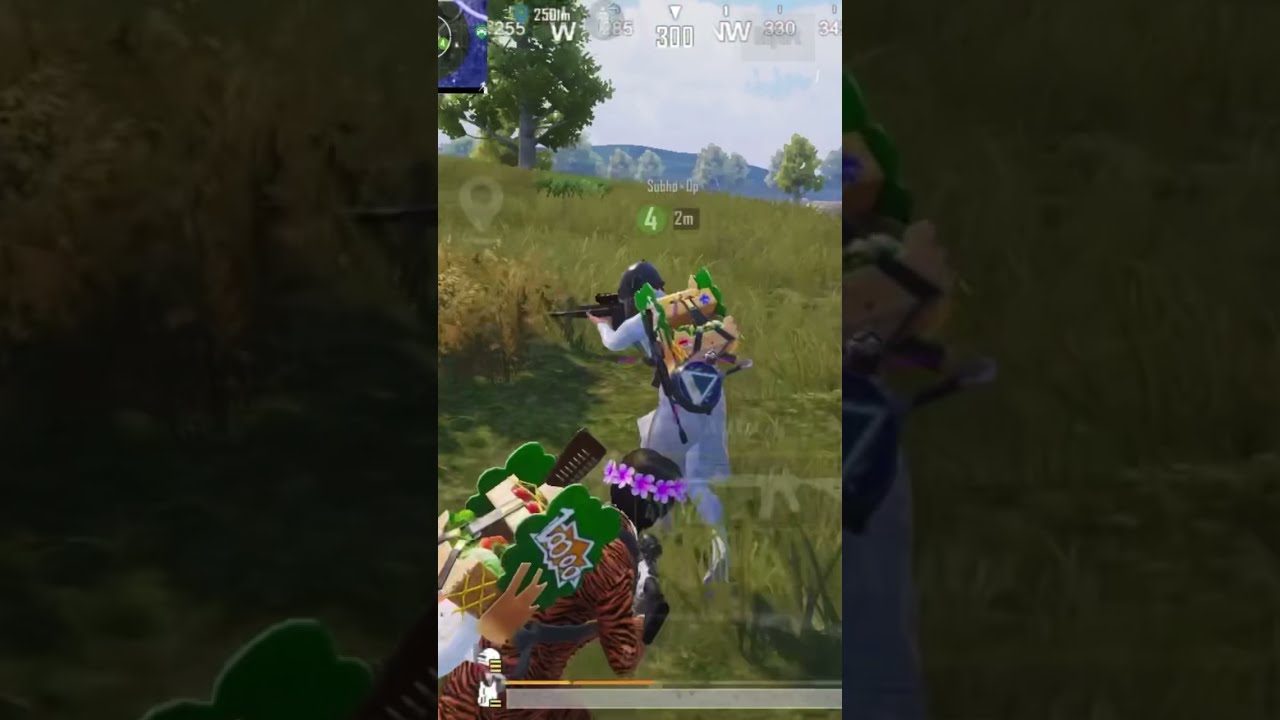The image showcases a scene from a video game, likely Fortnite, featuring two characters in a vibrant, natural setting. In the foreground, one character is dressed in a light lavender uniform or gown, wielding a black weapon aimed at the tall, green grasses. This character also sports a backpack that is gold with green accents. To their left stands another character, possibly female, adorned with a ring of purple flowers around a black head. This character wears a brown shirt with black lines, resembling a lion print, and possibly bears a green overlay. Both characters have backpacks, the second one featuring supplies like a spatula. The backdrop is rich with green-leaved trees, a bush with yellow or dead leaves, and a mountain range under a sky filled with white clouds and blue stretches. Text elements such as "255" and "W85" are visible at the top of the image, with the landscape sloping down as a grassy hill.